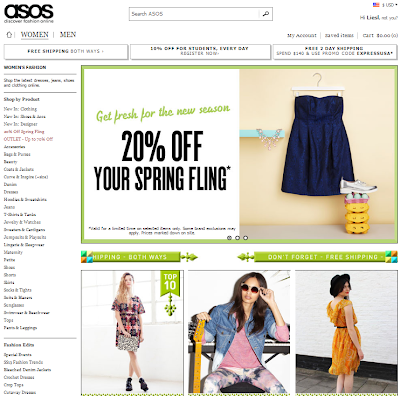The website for the clothing retailer Assos is showcased prominently. The Assos logo is placed in the top left-hand corner of the screen. Centered at the top is a search bar where users can enter their queries. On the far right-hand side are options to change the language or the country from which you wish to shop, accompanied by a login button.

Beneath the Assos logo are several main headings, including categories for women and men. Below these headings, larger banners promote offers such as 10% off certain items and free shipping. Along the left-hand side of the screen, there are additional headings for specific women’s or men’s clothing items.

The main body of the webpage features a prominent green border surrounding a central rectangle highlighting a special offer: "20% off your Spring Fling," written in black on a white background. Above this, green lettering announces, "Get fresh for the new season." To the right of this text, there is an image of a dress hanging on a hook, accompanied by a pair of training shoes displayed on a shelf.

Further down, three pictures feature women modeling various fashion styles, providing visual inspiration for potential buyers.